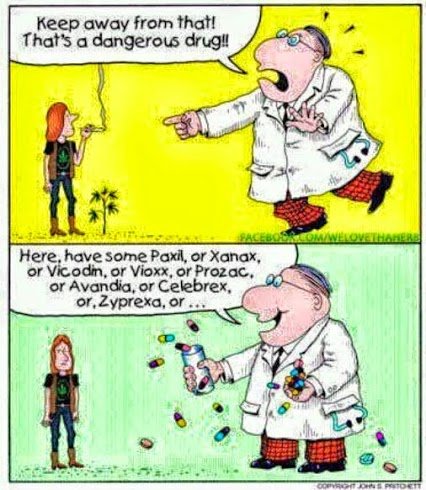The cartoon consists of two vertically stacked rectangular panels that are touching each other. The top panel has a bright yellow background, while the bottom panel features a pale green background with faint darker and lighter areas, giving it a somewhat striped appearance. On the right side of each panel stands a large, distressed-looking doctor wearing a white lab coat, red pants, black shoes, and small round glasses. He has a stethoscope hanging from his left pocket. The doctor occupies most of the right-hand side in both panels.

In the top panel, the doctor, whose mouth is wide open and who appears anxious with sweat marks near his head, is pointing at a hippie on the left side. The hippie, much shorter and skinnier than the doctor, with red hair, is smoking, and the smoke rises towards the doctor's speech balloon, which reads, "Keep away from that! That's a dangerous drug!!"

In the bottom panel, the doctor is smiling without any signs of anxiety. He holds a bottle in his right hand and a handful of spilling pills in his left hand, as if offering them. His speech balloon lists various prescription medications: "Here, have some Paxil or Xanax or Vicodin or Vioxx or Prozac or Avandia or Celebrex or Zyprexa or..." The hippie, now looking confused, stands with hands at his sides, facing the viewer. The plant he stood in front of in the previous panel, which resembled marijuana, and the marijuana leaf on his black shirt underline the contrast between the two figures.

The cartoon humorously critiques the discrepancy between the doctor's alarmed reaction to a natural substance and his casual, almost aggressive promotion of numerous man-made pharmaceuticals. The colors used throughout include yellow, green, white, red, black, and some hints of orange and blue.